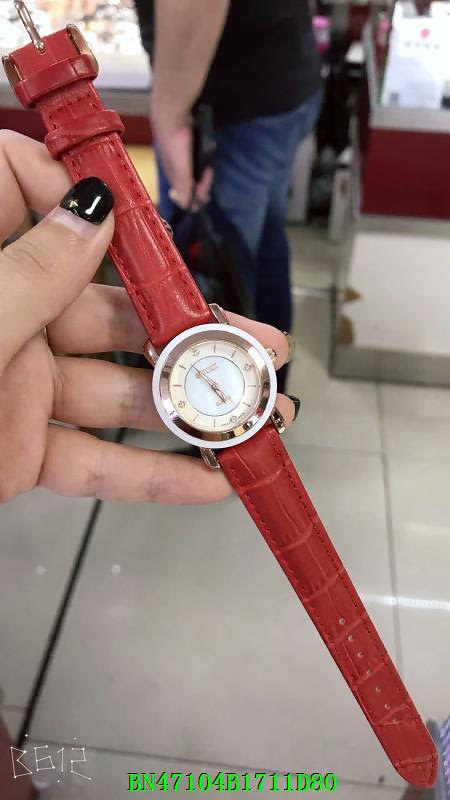In this vibrant and bustling public space, a woman’s hand, adorned with a striking watch, is prominently displayed, seemingly for sale. She stands against a backdrop of intricate tile flooring. The watchband is made of a reddish-orange, faux crocodile embossed leather, lending a touch of sophistication and texture. The watch face itself is an elegant combination of beige and white, embellished with gold numbers, a white border, and encased in a gold round frame, highlighting its luxurious design. Across from the woman, a man can be seen holding what appears to be a store package or perhaps a backpack. Attention to detail is evident in the lower part of the photograph, which features the letters "BN" followed by the sequence "4710, 4B17, 11D, 80." Additionally, the left corner showcases the identifier "B612."